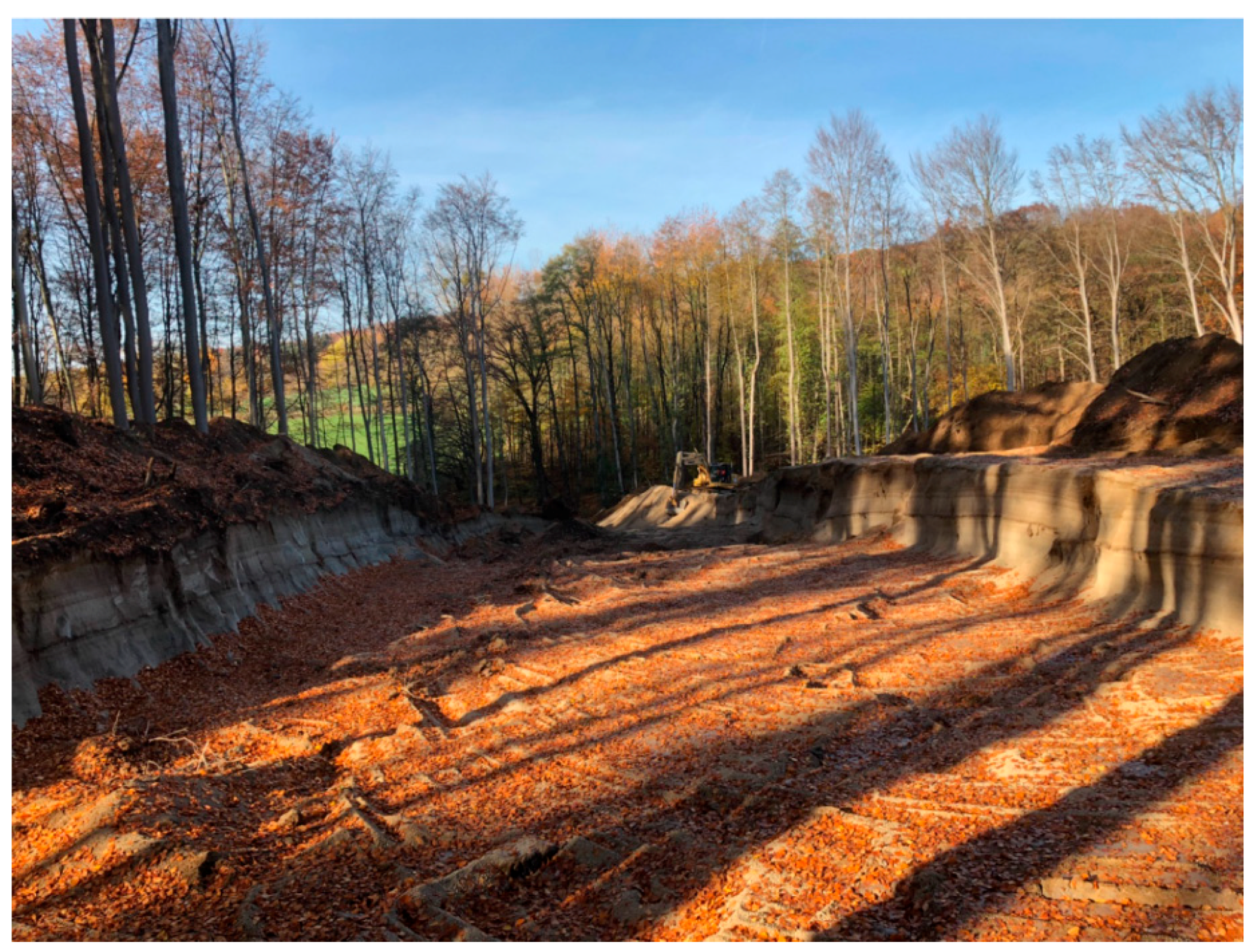This is an outdoor color photograph set during daylight, featuring a slightly rectangular composition. The primary focus of the image is a large, excavated trench or ditch area, approximately five to ten feet deep, stretching from the foreground to the horizon. This trench is lined with barren branches and trees showcasing autumnal colors of green, red, and orange, with scattered crumpled leaves covering the bottom. The edges are neatly uniform, flanked by two raised banks covered in dirt and leaves.

In the background, a row of trees stands tall, their foliage a mix of vibrant fall hues and some patches of bare branches. Further beyond, there's a distant view of hills adorned with autumn-colored vegetation, creating an intricate mosaic of green and amber. The blue sky above, decorated with white clouds, meets the tree line, completing the serene landscape. Amidst this picturesque setting, on the left side, a piece of construction equipment is visible, hinting at ongoing excavation work. Heavy shadows from the tall, thin trees fall across the ditch, enhancing the depth and texture of the scene. The overall composition captures the tranquil yet dynamic interplay of natural and man-made elements in their autumnal glory.